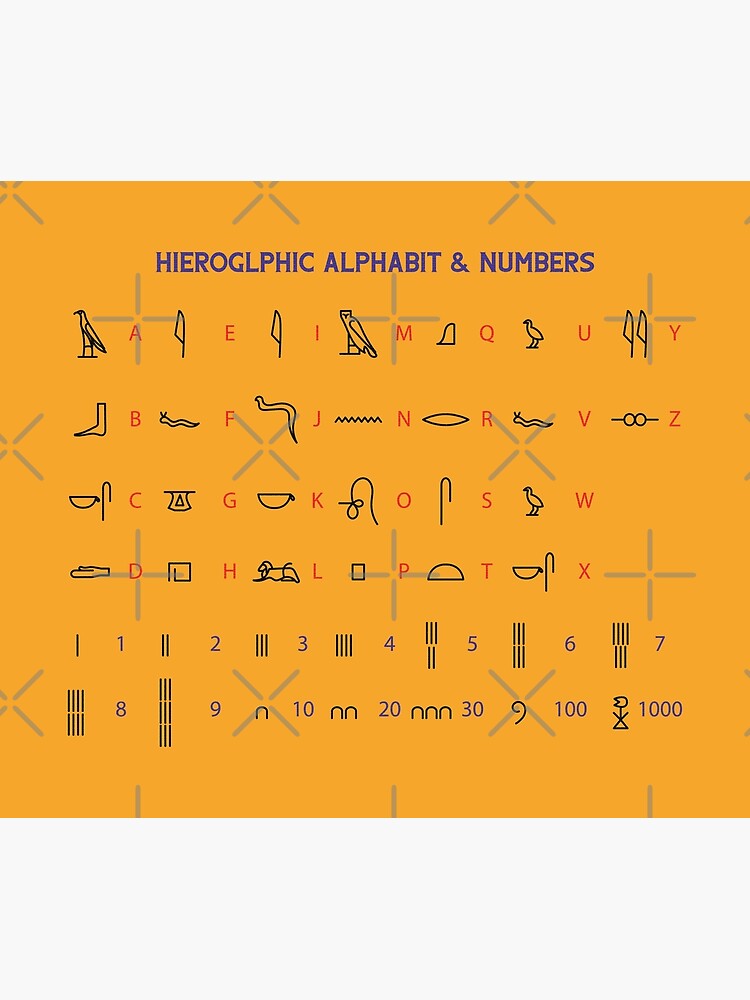The image is a digital illustration featuring Egyptian hieroglyphics alongside their Roman English letter equivalents. The background is orange with a decorative pattern of plus signs and crosses, and at the top, the title "Hieroglyphic Alphabet and Numbers" is written in purple print. Interestingly, "alphabet" is misspelled as "A-L-P-H-A-B-I-T."

The chart displays the hieroglyphic symbols in four rows. Each symbol is shown in black with its corresponding Roman letter written in red next to it. Some notable pairings include an A symbolized by a bird facing left, B by a leftward foot, C by a shepherd's hook and a cup, D by an open hand facing left, and so on through to Z, which resembles a set of glasses.

Following the alphabet, the image illustrates how numbers are represented through hieroglyphics. The numerals 1 through 9 are depicted using respective numbers of hash marks. The numeral 10 is represented by an N symbol, 20 by two Ns, 30 by three Ns, 100 is shown with a squiggly line resembling the number nine, and 1,000 by a flower-like symbol attached to a stick figure.

The image provides a detailed and visual explanation of how ancient Egyptian hieroglyphs correspond to modern English letters and numerals, enhanced by the contrasting orange background and distinct color coding for clarity.